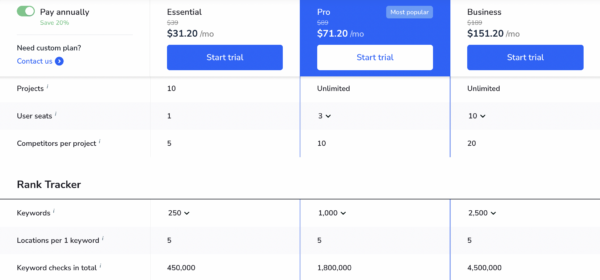The image is a screenshot of a web page displaying a pricing plan for a program. The background of the webpage is white. In the top left corner, there's a radio button labeled "Pay Annually, save 20%" that can be toggled on or off. The webpage is divided into four main columns: one for categories and three for different pricing plans labeled "**Essential**," "**Pro**," and "**Business**."

- **Essential Plan**: Priced at $31.20 per month, it includes a blue "Start Trial" button.
- **Pro Plan**: Priced at $71.20 per month, labeled as "Most Popular," and features a white "Start Trial" button.
- **Business Plan**: Priced at $151.20 per month, it also includes a blue "Start Trial" button.

On the left-hand side of the page, a list of features is displayed as follows:
- **Projects**: This shows "10" for Essential, "Unlimited" for Pro, and "Unlimited" for Business.
- **User Seats**: "1" for Essential, "3" for Pro, and "10" for Business.
- **Competitors Per Project**: "5" for Essential, "10" for Pro, and "20" for Business.
- **Rank Tracker Keywords**: "250" for Essential, "1,000" for Pro, and "2,500" for Business.
- **Locations Per One Keyword**: All plans offer "5."
- **Keyword Checks in Total**: "450,000" for Essential, "1.8 million" for Pro, and "4.5 million" for Business.

There is also a line that reads, "Need Custom Plan? Contact Us."

The pricing plan table is designed to help potential customers compare different subscription plans available under the annual payment option to determine which one best suits their needs.